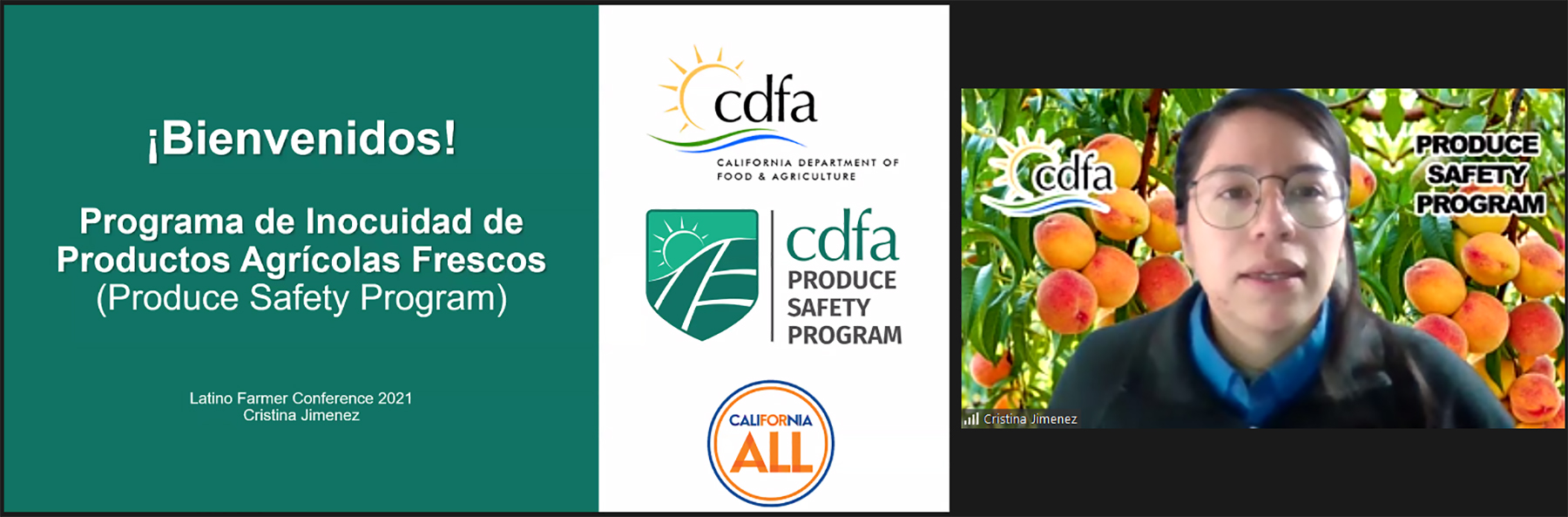The image is an informative flyer presented in a horizontal rectangle format, consisting of three distinct sections. The left portion features a dark aqua or blue-green background with text primarily in Spanish that welcomes viewers to the "Produce Safety Program," and includes a partial translation in English. This section also notes the "Latino Farmer Conference 2021" and mentions someone named Christina Jimenez. The central section, with a white background, showcases the logo of the California Department of Food and Agriculture (CDFA) and their Produce Safety Program. Notably, there is also a symbolic artwork of a sun included. The right portion of the image contains a photograph of a woman with dark, short hair and glasses, who appears to be of Spanish descent. She is standing in front of a tree lush with ripe peaches and green leaves. This section also displays the CDFA Produce Safety Program logo.